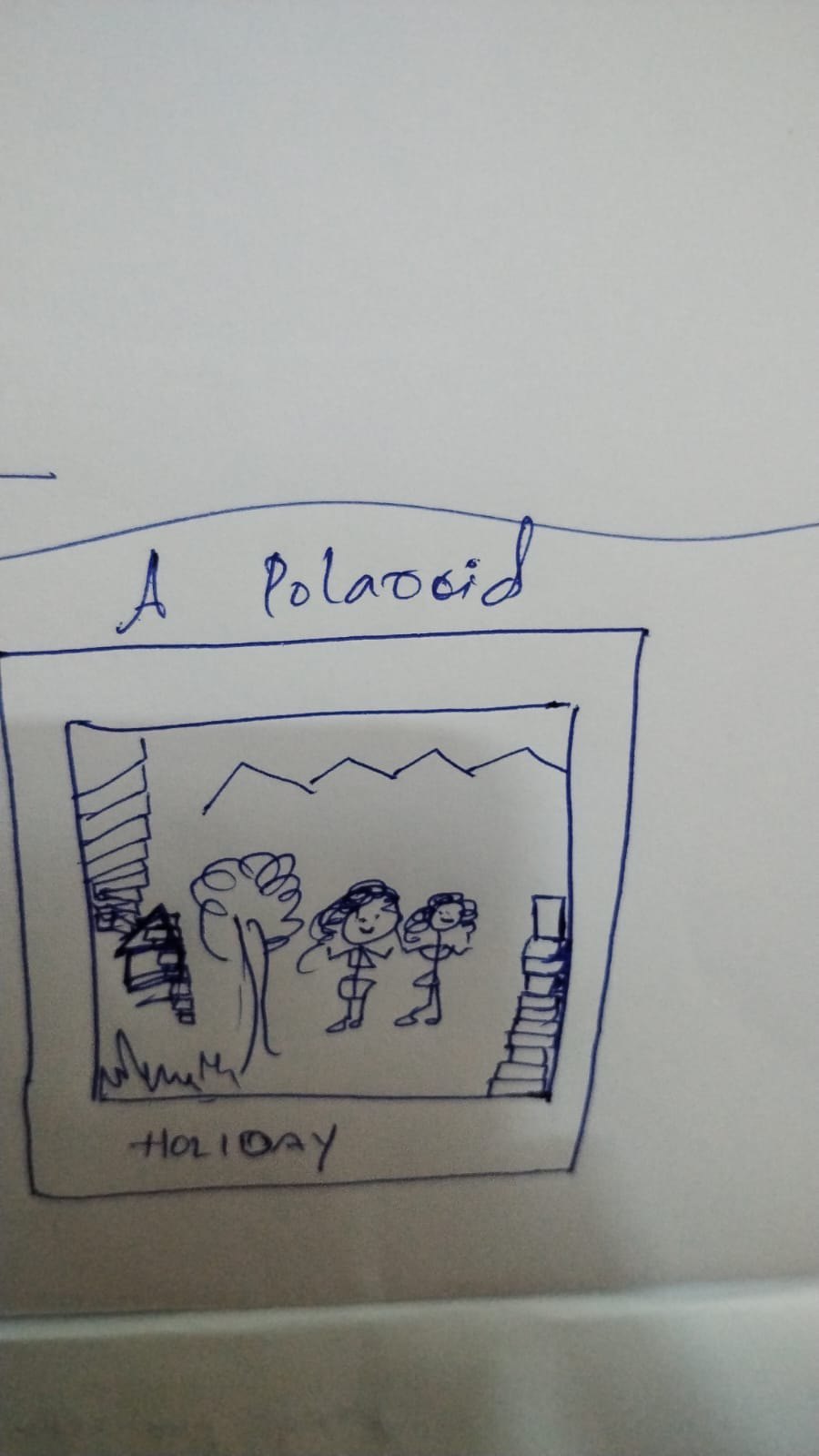This black-and-white ink drawing depicts two stick figure characters standing in a yard, smiling with dot eyes and a simple line for a mouth. Both characters have curly, long hair and are adorned with geometric shapes that suggest they are wearing swimsuits. Positioned to the right of a small, bushy-topped tree, the characters are set against a backdrop of a mountain range delineated by interconnected triangles across the top of the image.

The drawing is enclosed within a black square frame, with an additional square around it resembling a picture frame, all set against a white piece of paper. Text above the drawing reads "This is a Polaroid," while the word "holiday" is inscribed beneath it. This carefully composed work effectively captures a whimsical holiday scene.